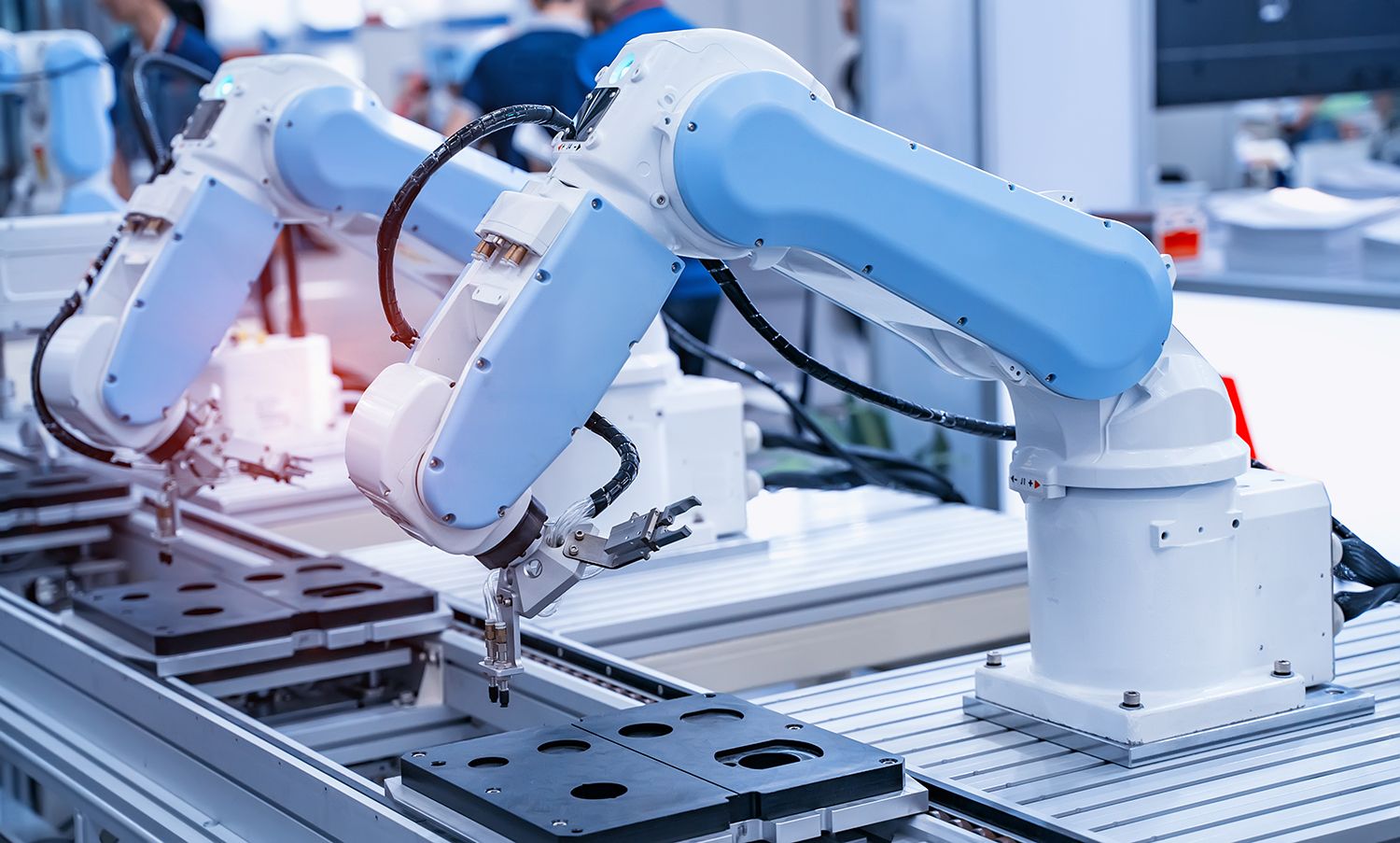In this image taken indoors, we see a highly technical machinery setup, situated in what appears to be a brightly lit and immaculately clean factory or laboratory. At the forefront, there are several robotic arms, each anchored by a sturdy cylindrical white base from which protrudes a large rectangular white box with attached cables. These cables snake into the elongated arms, which are predominantly white on top and light blue on the sides, with the arms bending downwards at pivot joints. The lower segments of the arms feature black wires attached, ending in intricate clamp-like mechanisms, resembling metal brackets with spinning heads designed for various tooling operations.

Below these robot arms, there's an assembly line positioned in the lower left side of the image. This conveyor belt system has two silver metal rails and transports rectangular blocks with black tops that have holes in them and silver plates underneath. These blocks are being attended to by the robotic arms, which are lined up on the right-hand side, diligently working over them.

In the background, the scene is slightly blurry but discernible – at least three individuals are standing around, possibly operating or monitoring the machinery. There are also tables with supplies scattered around, further indicating an industrial or laboratory environment. The entire room is characterized by its bright, white illumination and organized appearance.